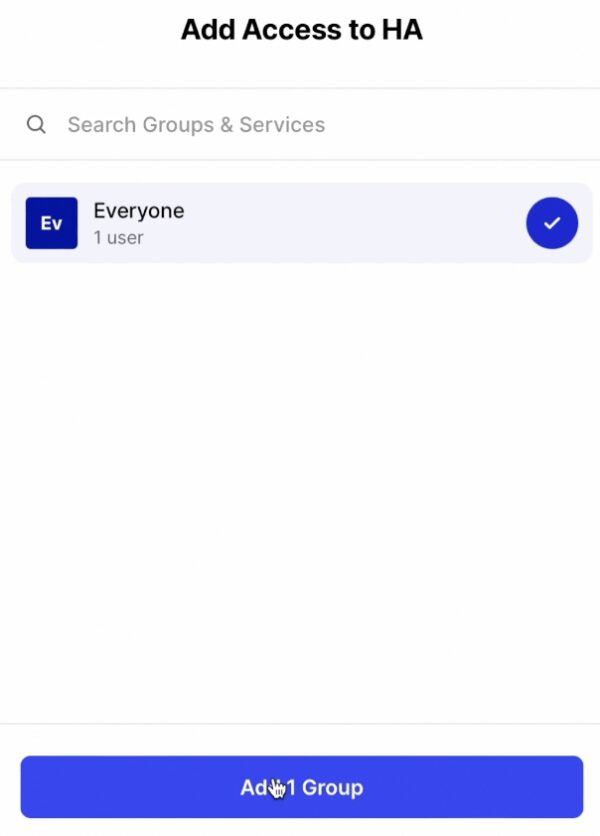This image is a screenshot from an unidentified source. At the top of the image, there is a heading that reads "Add Access to HA." Directly below the heading, there is a search bar accompanied by a black magnifying glass icon on the left side. Adjacent to the magnifying glass icon, the text "Search Groups and Services" is displayed. Beneath the search bar, there is a small dark blue square with the letters "EV" written in white. Next to this square, the word "Everyone" followed by "one user" is shown. To the right of this, there is a blue circle with a white check mark inside. At the very bottom of the image, within a dark blue rectangle, the text "Add One Group" is written in white, and a hand pointer icon hovers over the second "D" in the word "Add," indicating an imminent selection. The image contains no photographic elements or depictions of people, animals, birds, plants, flowers, trees, automobiles, motorcycles, bicycles, or airplanes.